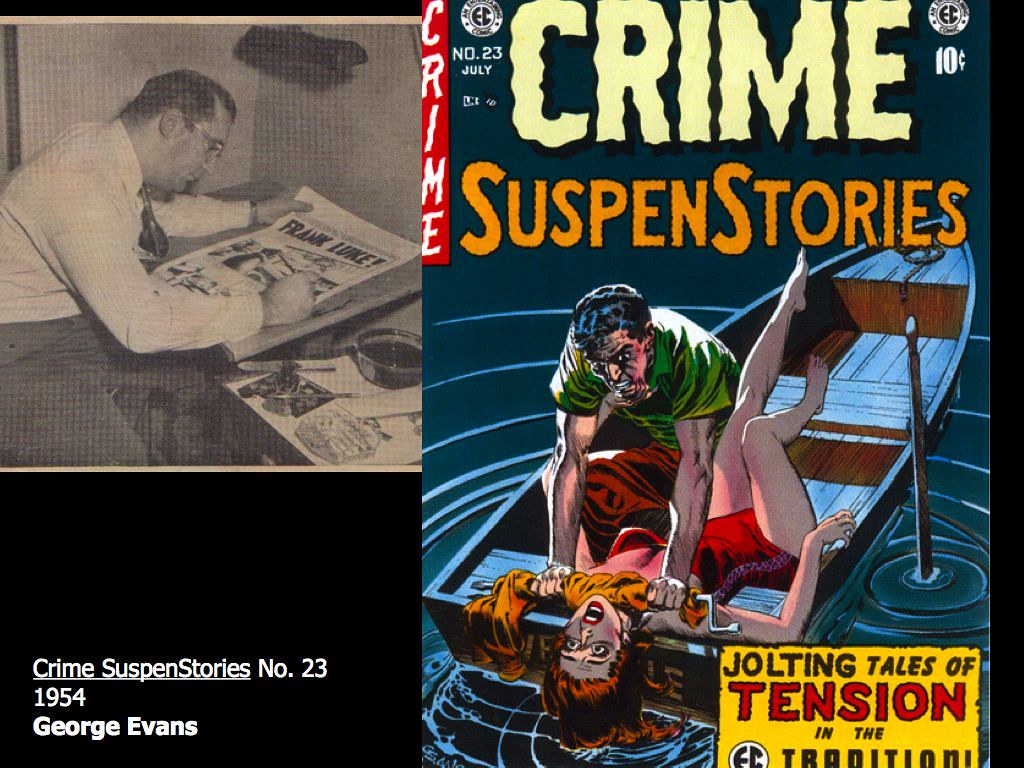The image depicts a juxtaposition of an illustrated comic book cover and a historical photograph. On the left side, there's an old black-and-white photograph of George Evans, identifiable by his dark hair, glasses, and white dress shirt, sitting and reading a newspaper. Below the photograph, a caption in white text on a dark background states: "Crime Suspense Stories No. 23, 1954, George Evans." The newspaper headline visible reads "Frank Lukey."

To the right of the photograph is the cover of Crime Suspense Stories No. 23, dated July 1954, priced at ten cents. The comic book cover features a dark blue backdrop resembling water. At the top left, a vertical red banner shows the word "CRIME" in white letters. The main title "CRIME SUSPENSE STORIES" is prominently displayed in large white and yellow letters, with "CRIME" in white against a dark background and "SUSPENSE STORIES" in yellow.

The central image on the comic book cover illustrates a dramatic scene: a man in a green t-shirt, with dark hair and an angry expression, holds a struggling woman in a red bathing suit. He appears to be restraining or choking her with his hands or possibly an orange cloth. The woman's head is tilted back over the edge of the rowboat, her hair trailing in the water, and her legs kicking upwards in panic. At the bottom right of the cover, there's a yellow box with text in black and red, stating "JOLTING TALES OF TENSION IN THE TRADITION OF…" but the final part is obscured.